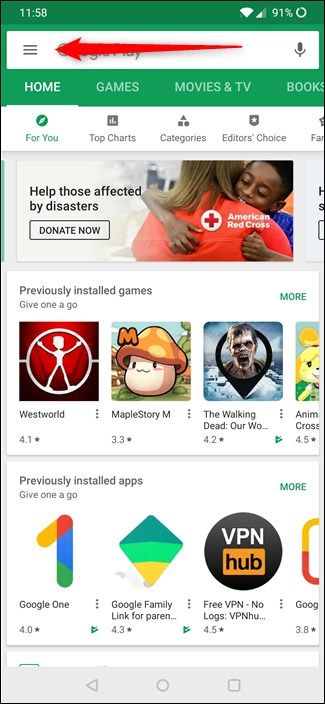The image is a screen capture taken from a mobile device, displaying an interface with a white background. At the top, there's a green horizontal frame housing a white search box. Below this frame, a series of selectable options are horizontally aligned: "For You," "Top Charts," "Categories," and "Editor's Choice."

Beneath these options, there's a touching photograph of a boy in a blue t-shirt embracing a woman in a red shirt. Printed on the back of the red shirt is the text "American Red Cross," and to its left in black font, the words "Help those affected by disasters. Donate now" are visible.

Further down, a section labeled "Previously Installed Games" encourages users to "Give one a go." Below this prompt, there are icons for various games, including one on the left depicting a man in a circle against a red square background. The text below this icon reads "Westworld."